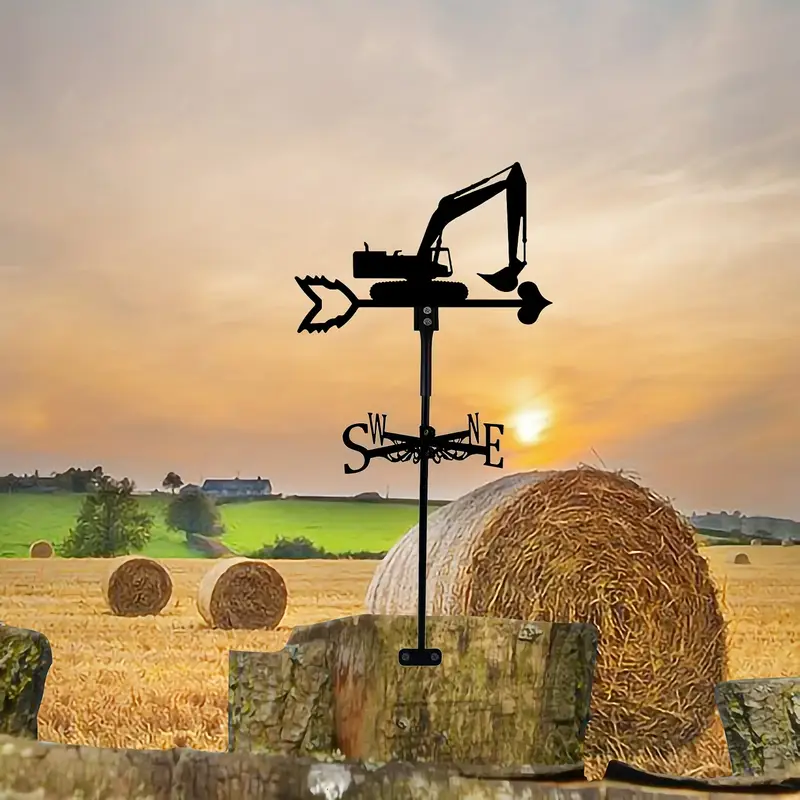In the foreground of this serene Midwestern hayfield, partially shrouded by semi-cloudy skies, a black, ornate weather vane stands out, mounted peculiarly on what appears to be a wooden fence or barrel. This weather vane features an arrow with a heart pointing to the right, as well as the cardinal directions—north, south, east, and west. The hayfield itself, recently harvested, showcases large rolls of brown hay scattered across its expanse. As the sun, either rising or setting, peeks through the clouds, it casts a gentle glow over the scene, creating a silhouette effect on the weather vane. Beyond the brown expanse of hay, a lush, green field stretches out, dotted with a few trees and culminating in a decently sized farmhouse near the horizon. The farmhouse, surrounded by more trees, anchors this peaceful countryside setting, though the mysterious placement and photorealistic quality of the weather vane suggest a potential composite image crafted from multiple photographs.